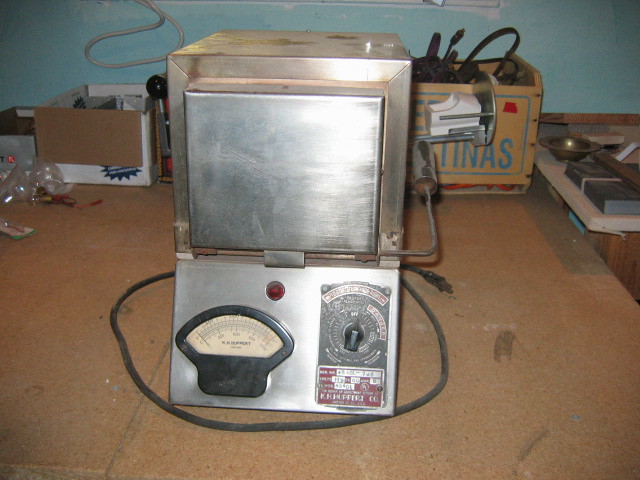This color photograph features an antique metal box-like device, seemingly an old kitchen appliance, possibly a kiln or an early model stove or oven. The apparatus is situated on a wooden counter with a cluttered background of a blue wall, assorted objects, and two boxes filled with electrical cords. The device itself is predominantly metal and has noticeable wear. 

The front of the device houses a small door, below which there is a control panel. On this panel, several dials and knobs are visible; one particularly distinctive knob could be turned to different settings, although the markings are too faded to clearly make out. Additionally, there's a lever on one side, resembling a slot machine handle, and an analog temperature gauge suggesting its function to regulate internal heat. The color scheme of the photo includes tones of brown, blue, white, and metallic hues, adding to the antique and nostalgic feel of the scene.